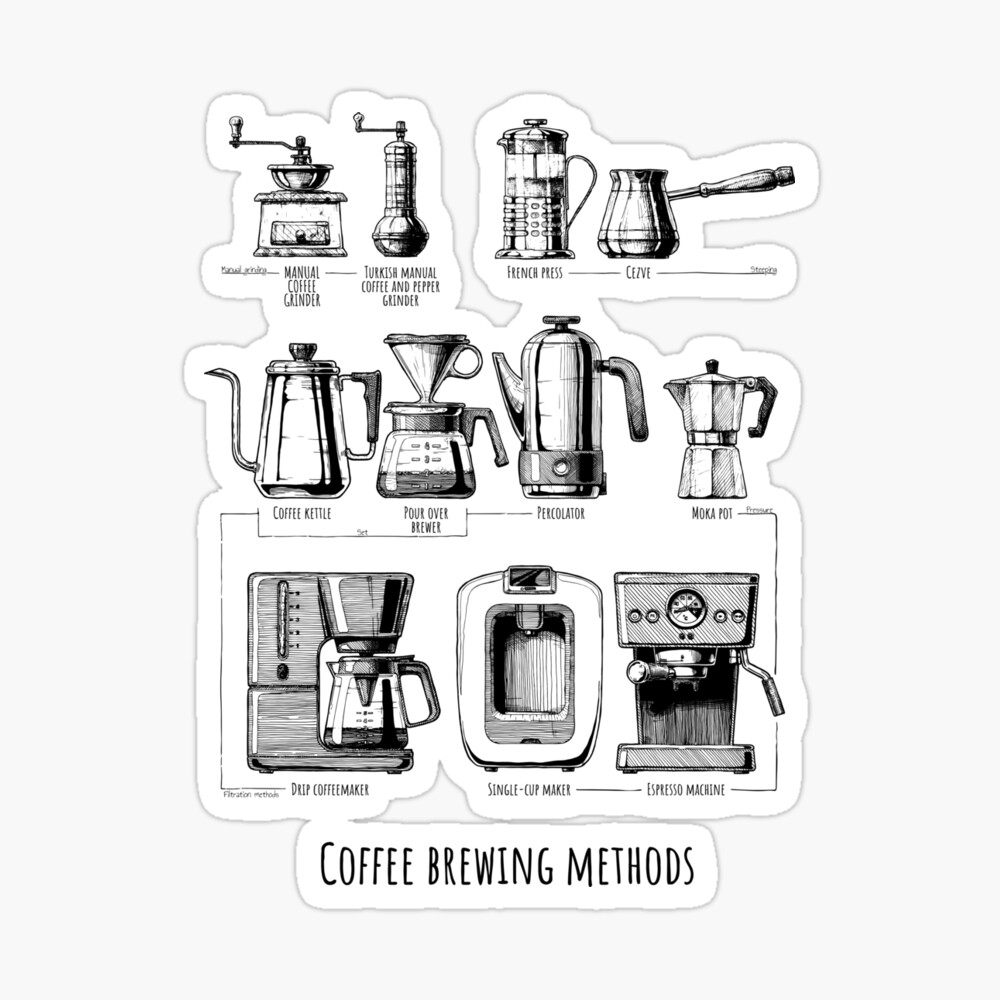This is a black and white illustration depicting various coffee brewing methods, outlined cohesively to resemble a sticker. The bottom of the image features the text "Coffee Brewing Methods" in bold, black letters. The illustration showcases 11 detailed sketches of different coffee makers arranged in three rows against a white background. In the top row, from left to right, there are depictions of a manual coffee grinder, a Turkish manual coffee and pepper grinder, a French press, and an additional item with partially legible text starting with "C". The middle row includes a coffee kettle with a long spout, a pour-over brewer, a percolator, and a mocha pot. The bottom row features a drip coffee maker, a single cup maker, and an espresso machine. Each device is labeled, and intricate lines adorn the sketches to subtly connect some of the devices. The entire image is set against a soft, off-white matte background.